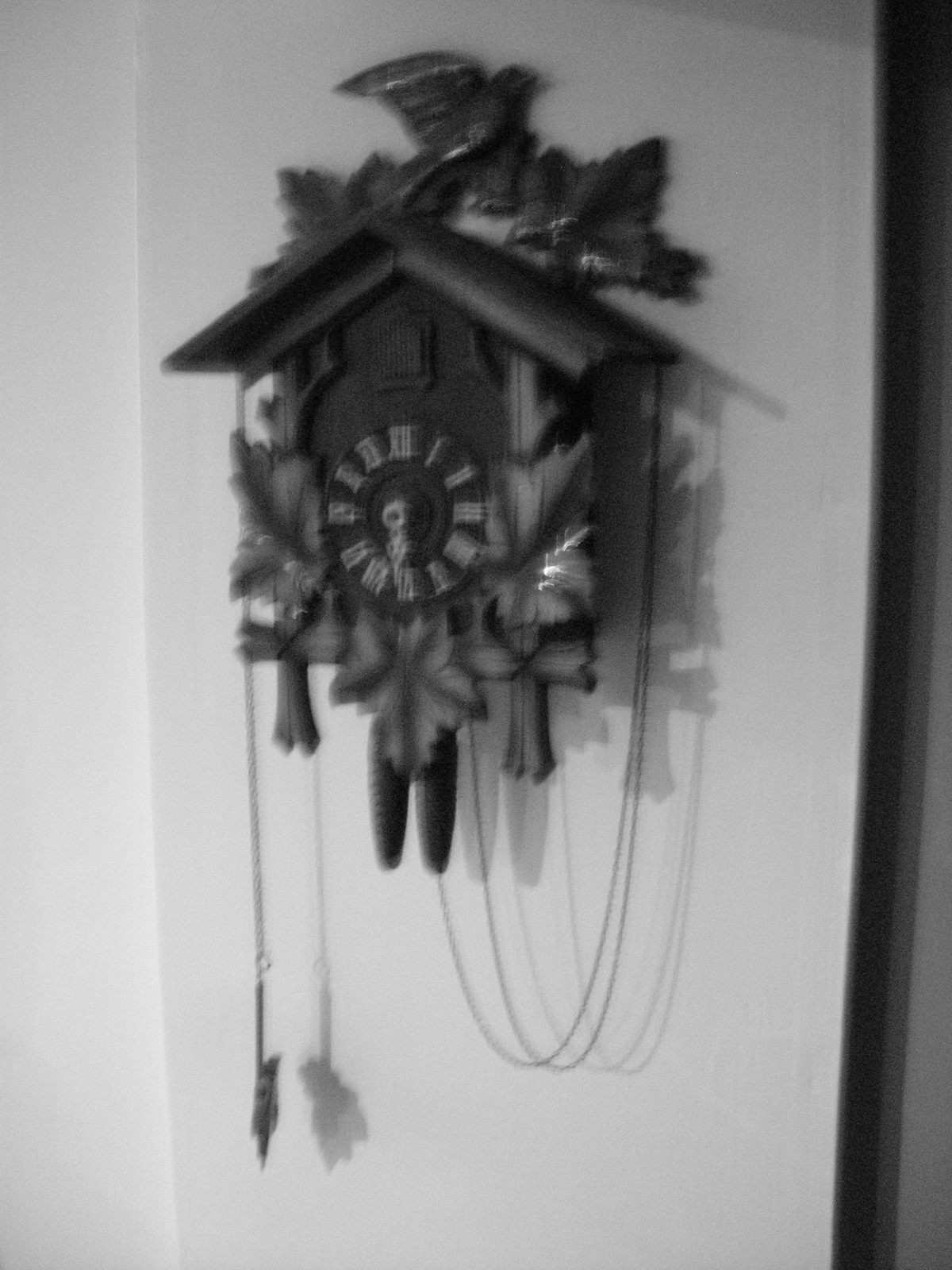This is a photo of a traditional Bavarian-style cuckoo clock hanging on a plain white wall. It appears to be an antique, likely made from wood sourced from German forests. Although the photo is in black and white and somewhat blurry, the clock's intricate details are still discernible. The clock is designed to resemble a small house with a gable roof, above which is a wooden carving of a bird with a wide wingspan, appearing to take flight. The face of the clock features Roman numerals and is surrounded by elaborately carved leaves and flowers, all painted black. Above the clock face, there is a small trapdoor from which the iconic cuckoo bird would traditionally emerge to announce the hours. Hanging below the clock are two weights on chains, which help power the clock's mechanisms, along with an additional unknown item on the left-hand side. The hands of the clock are white, providing a stark contrast against the black face, contributing to the clock's ornate and detailed appearance.